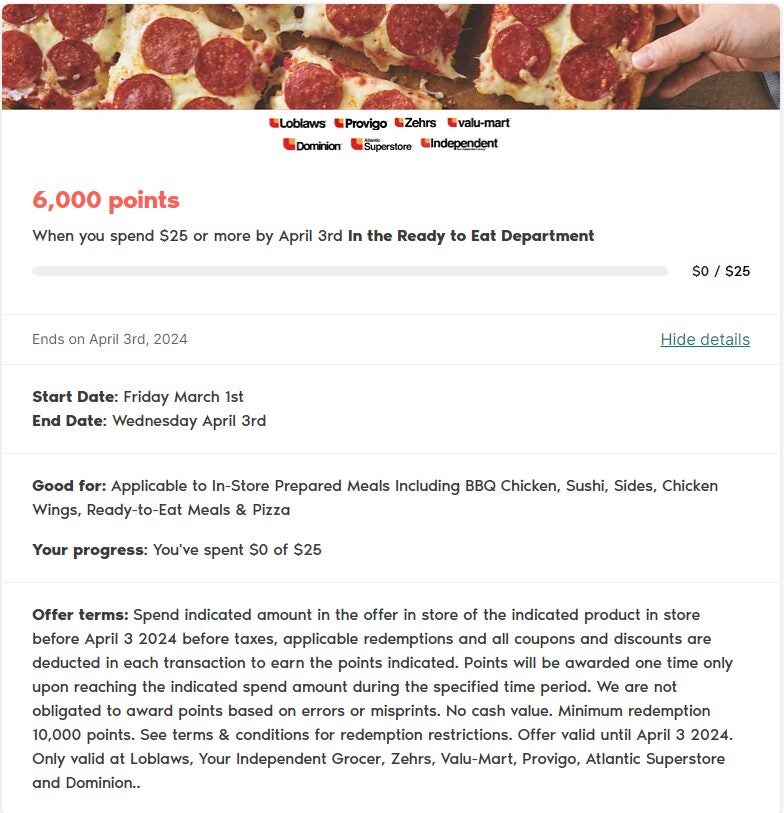Promotional Offer Details for Pizza Restaurant:

Earn 6,000 points when you spend $25 or more in the "Ready to Eat" department by April 3rd! This promotion begins on Friday, March 1st, 2024, and ends on Wednesday, April 3rd, 2024. 

Eligible purchases include in-store prepared meals such as barbeque, chicken, sushi, sides, chicken wings, ready-to-eat meals, and pizza. 

To qualify, spend the specified amount of $25 before taxes and after all applicable coupons and discounts. Points will be awarded only once during the promotional period. Note that this offer has no cash value and requires a minimum of 10,000 points for redemption.

Be sure to read all terms and conditions regarding restrictions. Don't miss out on this fantastic limited-time offer!